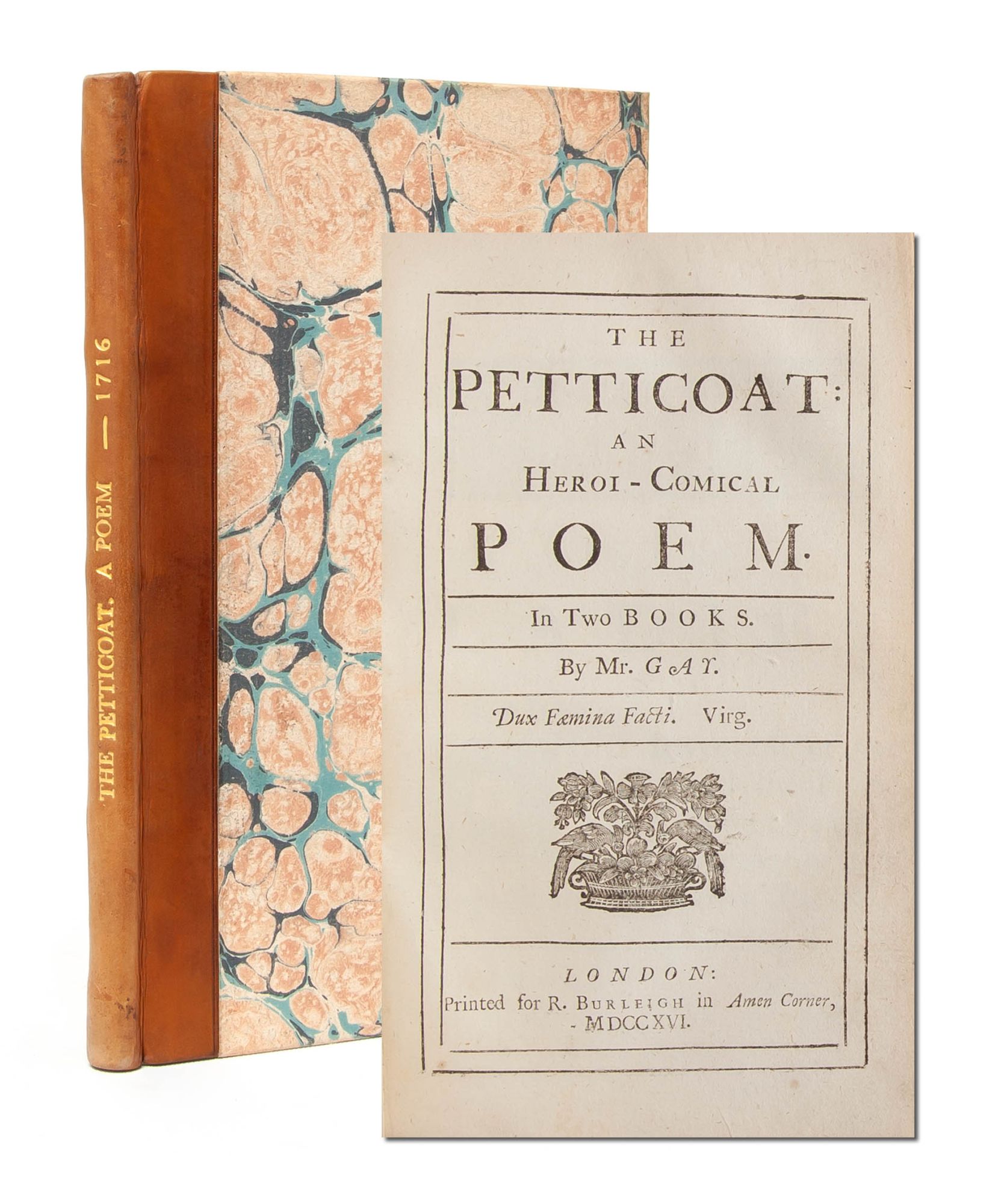This detailed up-close photograph showcases an antique book titled "The Petticoat, A Poem, 1716," positioned behind what appears to be its title page. The book has a brown leather spine with gold print that reads "The Petticoat, A Poem, 1716." The cover features a marbled design in orange-beige with blue and dark blue veins. In front of this book lies an aged, browned title page, which reads "The Petticoat, An Heroic Comical Poem in Two Books, by Mr. G.A.T., Dux Femina Facti, printed in London for R. Burleigh at Amen Corner." The title page also includes an intricate black and white illustration of two birds pecking at a pot of flowers, emphasizing its historical and delicate nature.